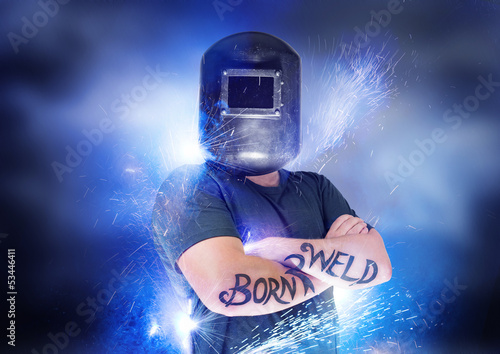This rectangular image, approximately 4 inches wide and 3 inches tall, features a male welder with his arms crossed. He is wearing a dark navy short-sleeved shirt and a black welder's hat with a glass slot obscuring his face. His forearms are adorned with tattoos: the right arm bears the word "Born" and a symbol, while the left arm displays "Weld" with an additional symbol. When his arms are crossed, the tattoos align to form the phrase "Born to Weld," incorporating the number 2. The background is alive with flying sparks, set against purplish, black, and white-gray hues. The words "Adobe Stock" appear repeatedly in a transparent pattern across the image, and the lower left corner prominently displays the number 53446411.